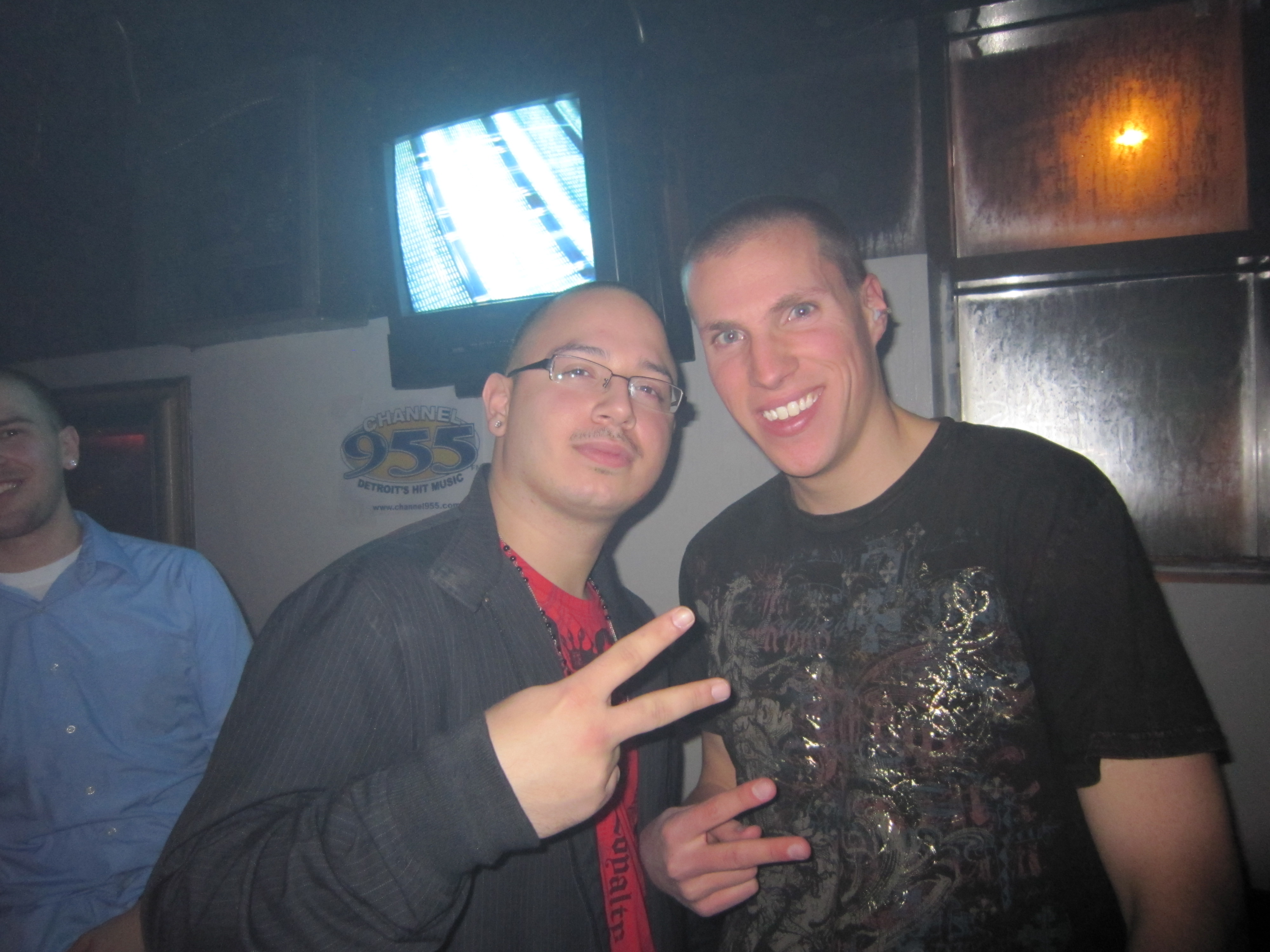In a lively bar setting, two men are posing together for a photo, both flashing peace signs. The man on the left is bald with a closely shaved head, wearing glasses, and dressed in a black jacket over a red t-shirt. He has a thin mustache and an ear piercing. Illuminated by the camera flash, the details of his attire and appearance are clearly visible, including a Channel 955 sign nearby and a vintage tube TV mounted above his head, its screen glowing. Next to him, the slightly taller man on the right has very short, thinning hair and is beaming a big smile. He has blue eyes, an earring in his left ear, and is clad in a black t-shirt adorned with a shiny silver, gold, and gray graphic design featuring a tree and white crosses. The warm, bustling atmosphere of the bar is palpable behind them. To the far left, partially visible, another man in a blue button-up shirt over a white t-shirt can be seen smiling, adding to the camaraderie captured in the photo.